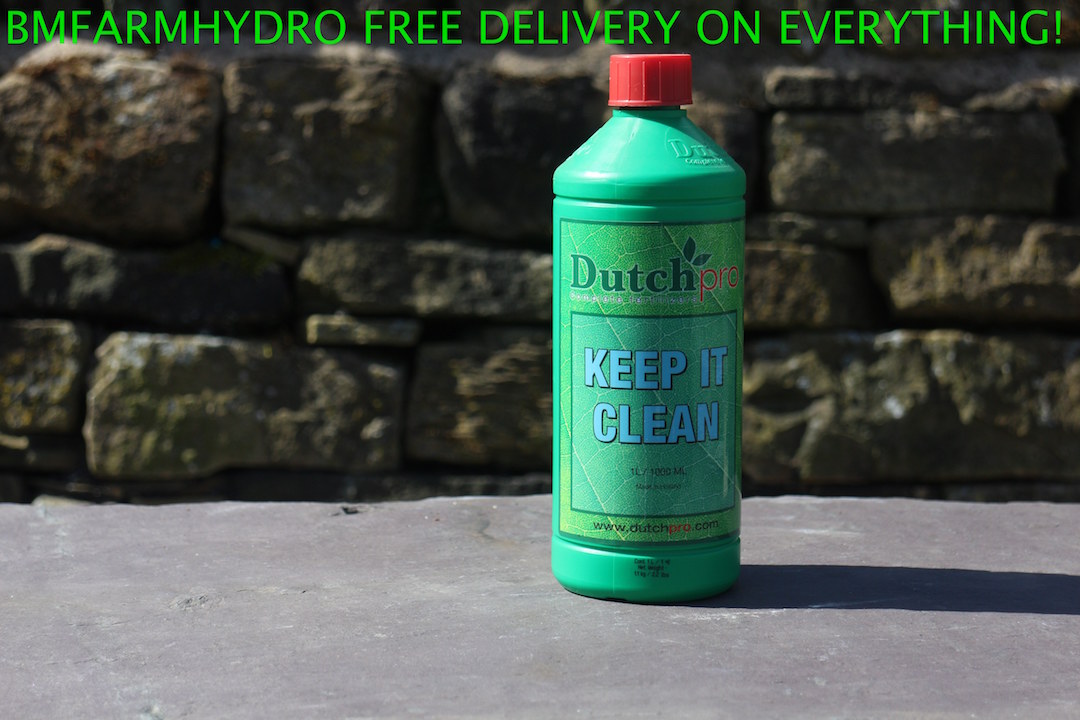The photograph features a green bottle prominently displayed on a concrete surface, possibly a table or sidewalk, with a brick wall serving as the backdrop. This bottle, which has a red cap, is decorated with green lettering that reads "Dutch Pro" and "Keep it clean," suggesting it is a cleaning or maintenance product related to hydro farming. Above the bottle, in the photograph, bold green text proclaims, "BM Farm Hydro, free delivery on everything!" The bottle’s shadow is cast to the right side, adding depth to the scene. This meticulously arranged ad aims to promote the Dutch Pro product, highlighting its availability and the free delivery service offered by BM Farm Hydro.